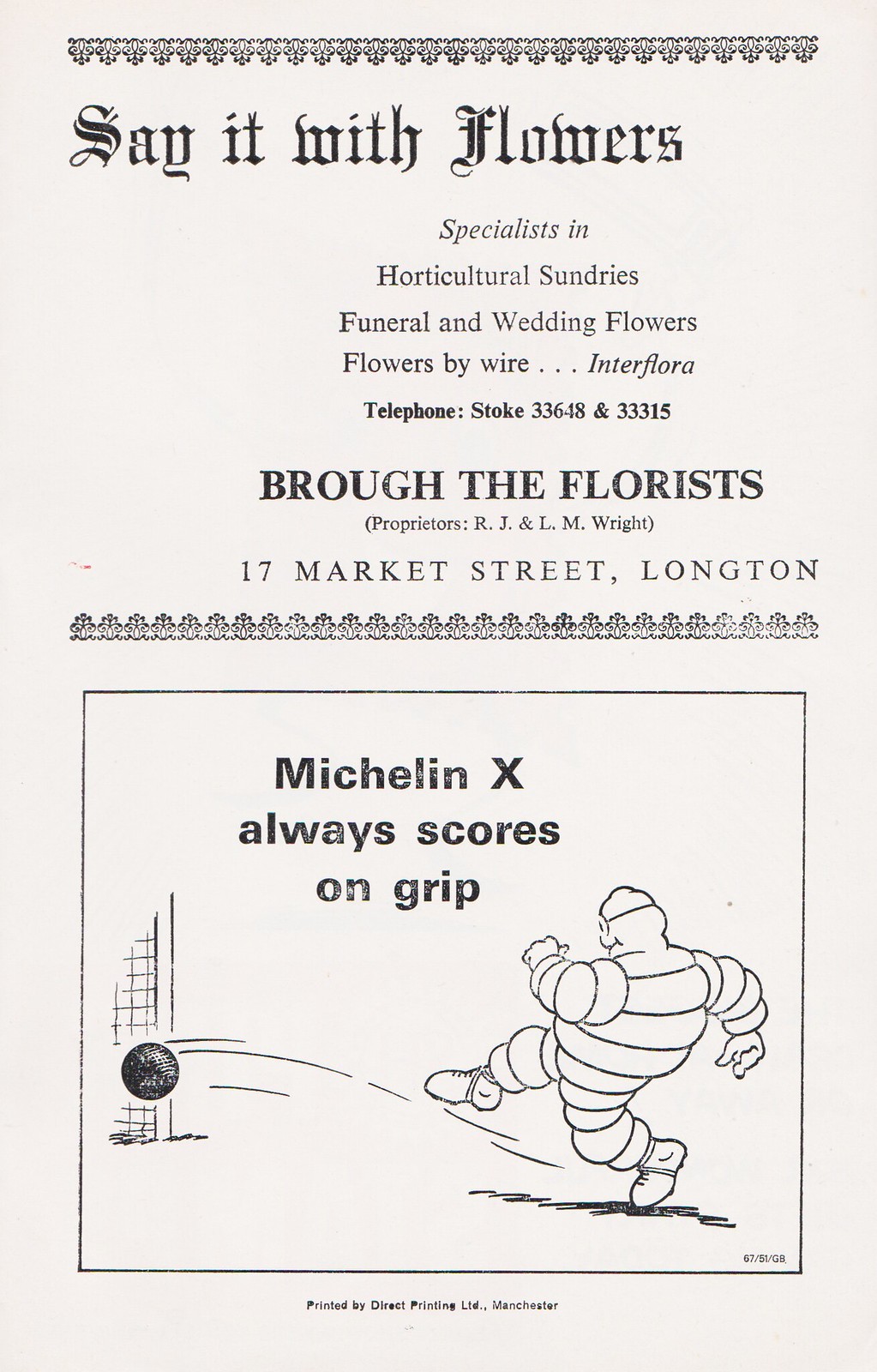The image is a white postcard featuring elements from old advertisements. The top section showcases elegant, vintage-style script reading "Say It With Flowers," followed by a typewriter-style font listing "Specialists in Horticulture Sundries, Funeral and Wedding Flowers, Flowers by Wire, Interflora. Telephone: Stoke 33648 and 33315. Bro the Florists, Proprietors R.J. and L.M. Wright, 17 Market Street, Longton." The bottom section contains a hand-drawn cartoon of the Michelin Tireman, identified as the Michelin Man, kicking a soccer ball into a net, with the slogan "Michelin X Always Scores on Grip" prominently displayed. The entire composition suggests it is a photocopy of an aged flyer or advertisement page, retaining a crisp appearance despite its vintage origin.